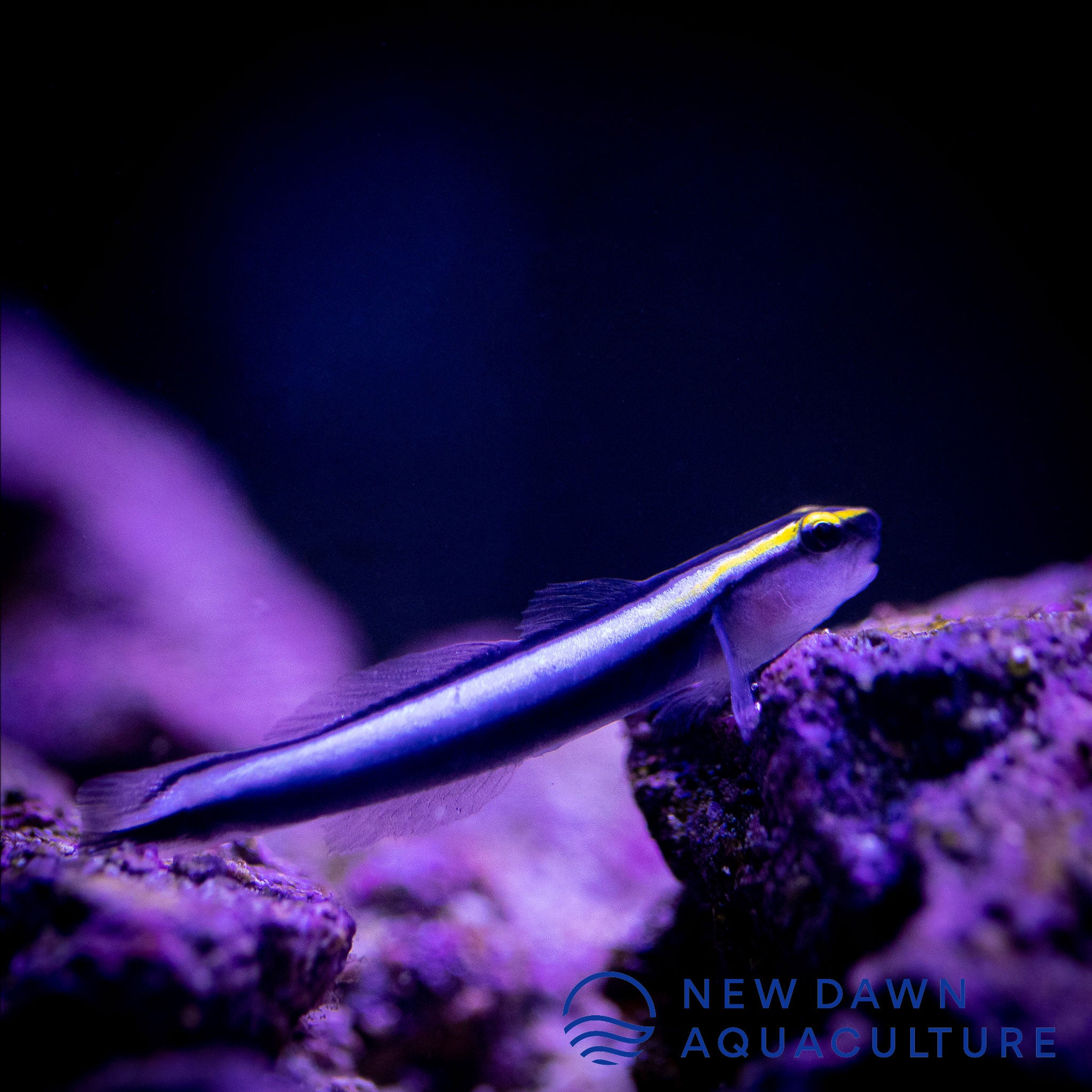The image features a detailed, close-up view of a long, slender fish with a shimmery palette of dark blue, silvery-blue, and purplish hues. The fish, which has distinct, small fins reminiscent of feet near its front and large, reflective eyes with a touch of yellow, stands out against a dark background that transitions from a nearly black-blue at the top to a lighter blue and then purple towards the bottom. Surrounding the fish are glistening black-and-white rocks that also carry a purplish tint, likely due to the photograph's lighting. In the bottom right corner, the New Dawn Aquaculture logo is visible, featuring a round circle with wave patterns in the lower half, accompanied by their name in blue type.